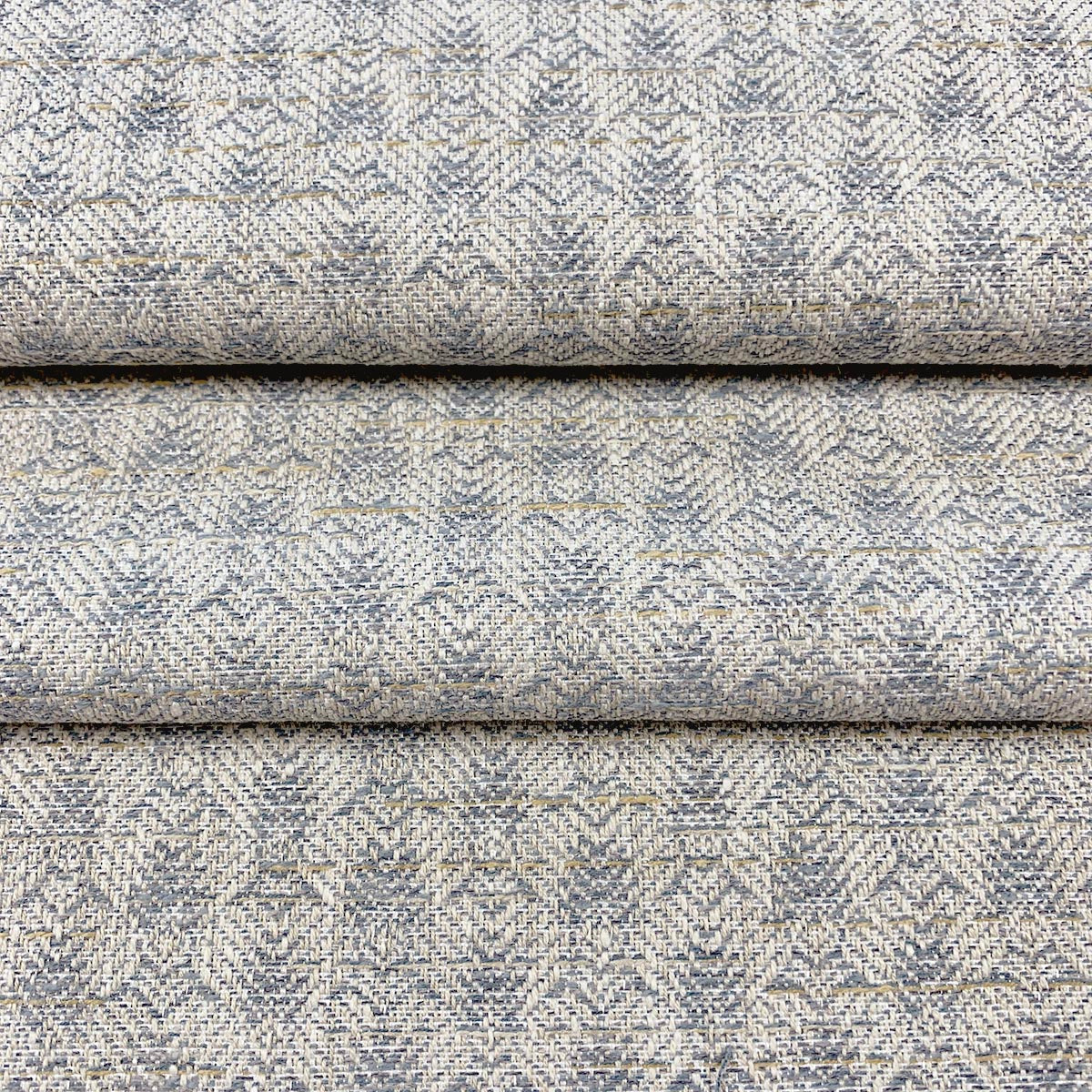The image features three pieces of fabric, all made from the same material and in the same color. The fabric is stacked in a way that resembles steps rather than being flat on top of one another. They have a woven pattern with a palette that includes shades of blue, gray, and white, and also includes off-white and slight tan designs. The fabric exhibits a design of closely set, pointed shapes running across its surface, reminiscent of a burlap texture. This detailed pattern gives the appearance that the fabric could potentially be used as rugs, carpeting, or possibly blankets. The overall color tone of the fabric resembles light stone gray, with bluish hues interspersed throughout.